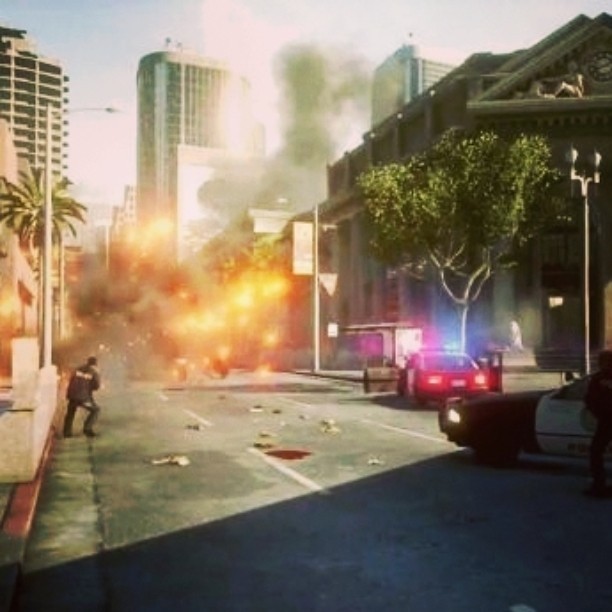The image, which appears to be a computer-generated scene from a video game, depicts a chaotic urban street setting. In the foreground, multiple police cars are parked haphazardly with their doors open and lights flashing, suggesting a recent arrival to an emergency. The street is littered with pieces of debris possibly from an explosion, and there's a hint of blood on the ground. The scene is dominated by a large, fiery explosion further down the street, billowing gray smoke skyward. The explosion is intense, casting a bright yellow glow amidst the dusky environment. A policeman stands near his vehicle on the right side of the image, while another figure, potentially a firefighter or another officer, is visible to the far left. The background showcases tall buildings typical of a cityscape, including a notable museum-like structure adorned with sculptures and a clock face, supported by large pillars. Amidst the scattered trash and hectic scenario, the weather remains paradoxically clear and sunny, highlighting the palm tree and other street trees lining the street.